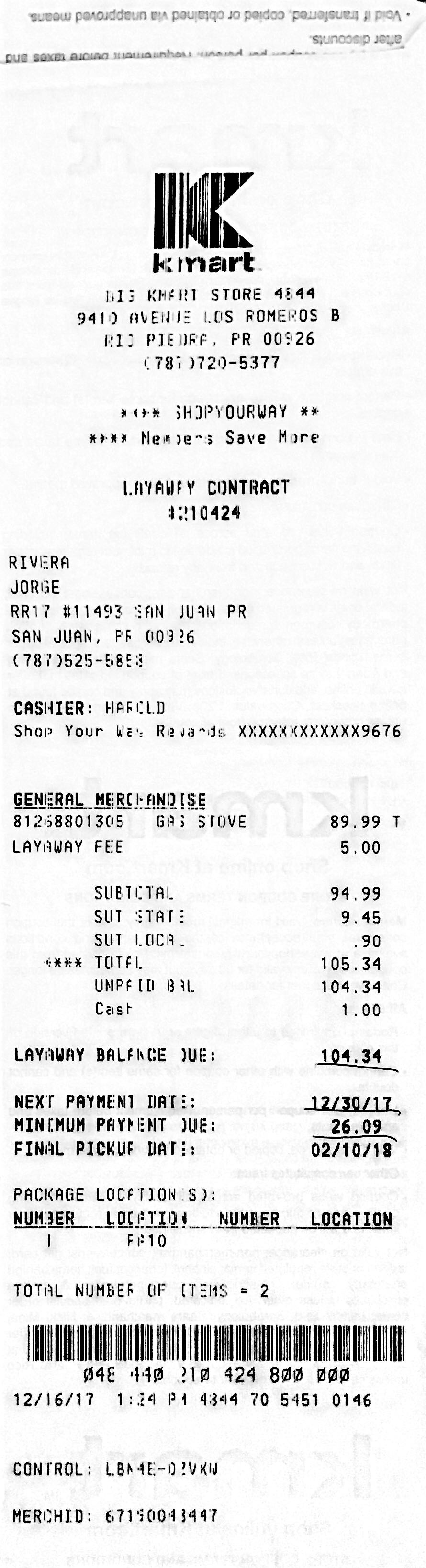This image is a scanned and slightly blurry photograph of an old, faded Kmart receipt. The receipt is from Kmart store number 4844, located on Avenue Los Romeros in San Juan, Puerto Rico. The receipt, dated December 16, 2017, details a layaway contract for a gas stove priced at $89.99, with a layaway fee of $5.00. After additional taxes and fees, the total amount due was $104.34. The customer's name is Jorge Rivera, and the cashier handling the transaction was named Harold. The next payment of $26.09 was due on December 30, 2017, with the final pickup date set for February 10, 2018. The receipt also includes a partially legible 787 phone number and mentions "Shop Your Way" rewards.